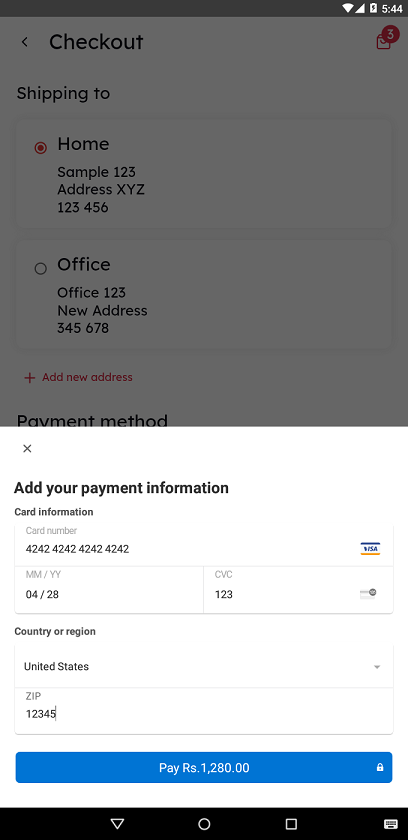This screenshot captures a phone screen where someone is in the process of completing an online payment. The top half of the screen is slightly dimmed with a transparent gray overlay, suggesting it is part of an active modal or pop-up window. At the very top of the screen, you can see the phone's status bar: the Wi-Fi connection icon shows it is connected, the battery icon indicates a full charge, and the time reads 4:55 PM.

Within the gray overlay section, there's a "Checkout" label accompanied by a black left-pointing arrow. In the top-right corner, there's a red notification icon with a square checkmark and the number three, indicating three unread notifications.

Further down, the section for selecting a shipping address is shown. Currently, the "Home" address is selected, marked with a red dot. The home address listed is "Sample 123 Address, XYZ 123456." An alternative address option labeled "Office" is available but unselected, showing "Office 123, New Address, 345678" next to a grayed-out dot. Beneath these options is a red plus sign for adding a new address.

Below this, the screen is cut off where it mentions the "Payment Method." Transitioning to the lower portion, set against a white background, is an "X" button in the top-left corner, probably to close the screen. It prompts the user to "Add payment information," including fields for "Card Information," "Credit Card Number," "Month and Year," "CVC Code," "Country or Region" (with "United States" selected), and "ZIP Code." At the bottom of the screen, a blue button with white text awaits for the user to "Pay RS-10280."